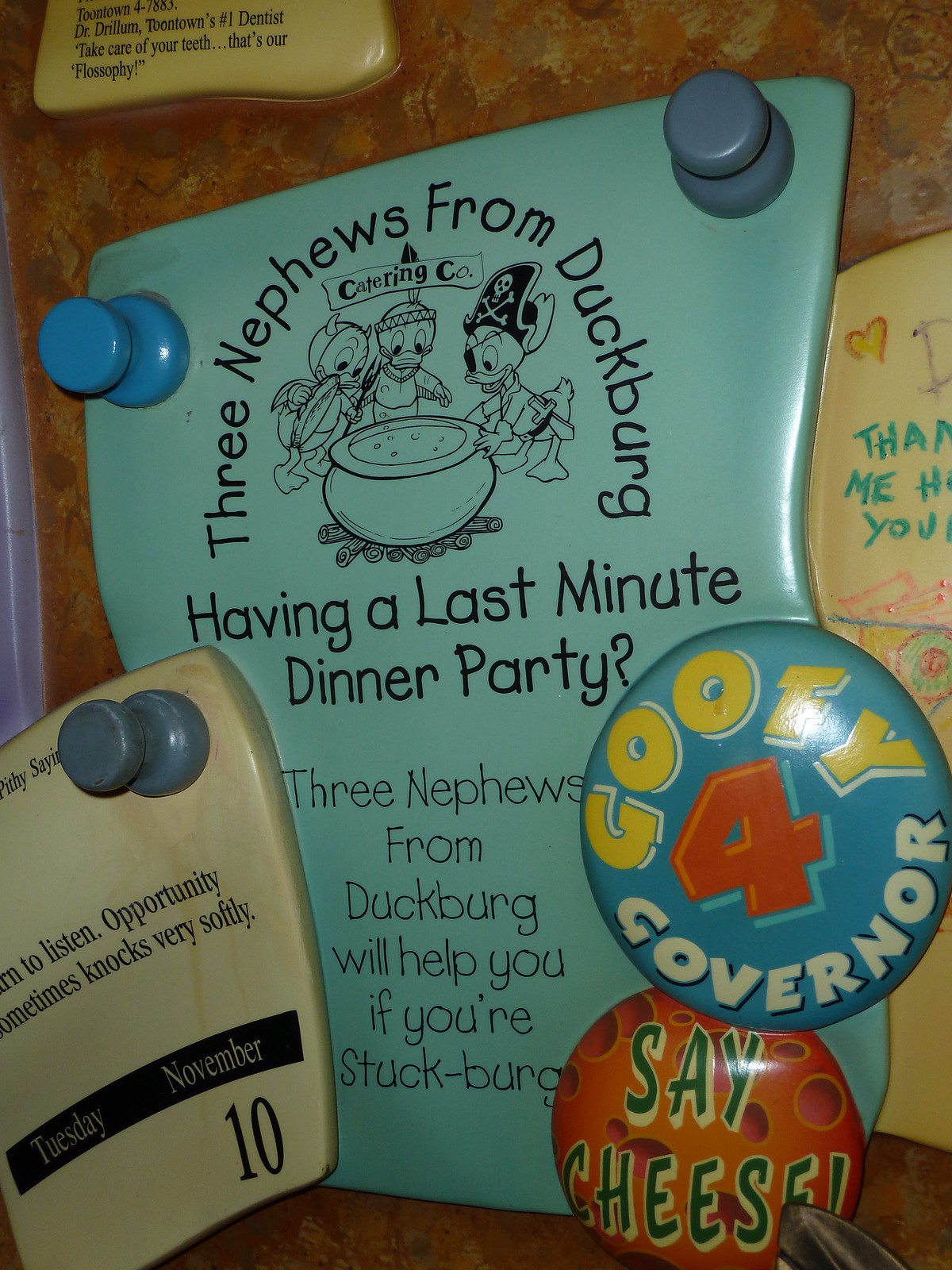The image depicts a bulletin or cork board adorned with various pins and buttons, adding a nostalgic, childlike charm to the scene. Dominating the board is a wavy, light blue ceramic piece with the inscription "Three nephews from Duckburg," referencing Disney characters Huey, Dewey, and Louie. These three ducks are illustrated around a cauldron in Halloween costumes—one dressed as a devil, one as a Native American, and one as a pirate. Below the illustration, the text reads, "having a last-minute dinner party. Three nephews from Duckburg will help you if you're stuck-burg." Also on the board is a round pin that says "Goofy for Governor" and another that reads "Say Cheese." The date "Tuesday, November the 10th" is visible on the ceramic piece, along with the phrase "Opportunity sometimes knocks very softly."